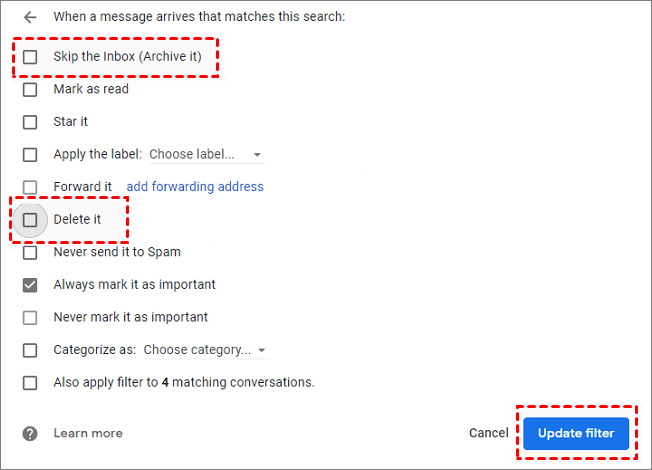A detailed image description for the provided caption:

This image depicts a section of an email filtering settings interface commonly found on a computer or smart device. The background appears to be transparent, utilizing the white of the underlying screen. A thin black border outlines the square setup interface.

At the top left, there is a left-facing arrow followed by the text "When a message arrives that matches this search:". Below this text, several checkbox options with corresponding actions are displayed:

1. "Skip the Inbox (Archive it)" – This option is emphasized with a dashed red border around it.
2. "Mark as read"
3. "Star it"
4. "Apply the label: choose label" – Accompanied by a downward-pointing arrow indicating a dropdown menu.
5. "Forward it to:" – Followed by a blue link text "Add forwarding address."
6. "Delete it" – This option is also highlighted with a dashed red border.

Surrounding the entire square is a light gray circle, adding further distinction to the section.

Continuing down the list:
7. "Never send it to Spam"
8. "Always mark it as important" – This box is checked.
9. "Never mark it as important"
10. "Categorize as: choose category" – Again featuring a downward-pointing arrow for selection.

Additionally, there is an option "Also apply filter to # matching conversations" suggesting applicability to existing emails.

At the bottom left of the square, there is a small question mark icon linked to "Learn more" for further guidance. Moving towards the bottom right, there are two buttons: a "Cancel" button and a blue "Update filter" button with white text. The "Update filter" button is also outlined with a dashed red border, drawing attention to it.

The various elements such as checkboxes, dropdown arrows, and highlighted areas with dashed red lines and emphasized text are clearly distinguished to enhance the usability and understanding of the filter settings interface.